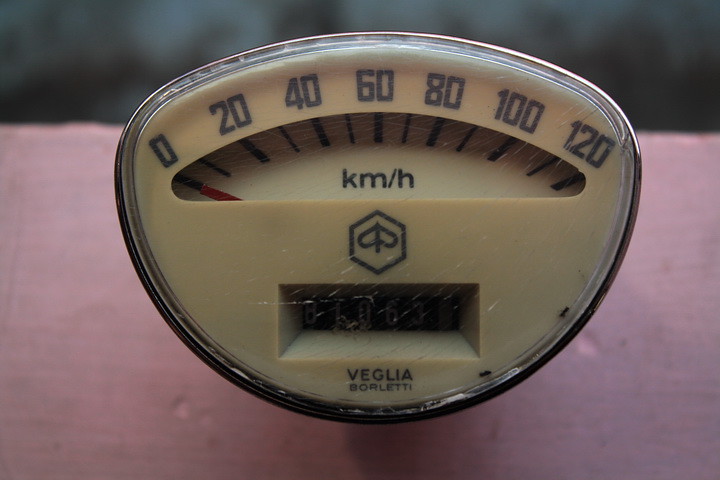This image features a uniquely designed speedometer with an elongated oval shape, where the bottom forms a U-like curve and the sides extend upwards to meet a wider top, making the overall shape resemble an elongated oval. The speedometer displays large numerical markings at the top, indicating speeds of 0, 20, 40, 60, 80, 100, and 120, with smaller intervals marked below for each 10-unit increment from 0 to 120. The smaller markings are labeled clearly for 10, 30, 50, 70, 90, and 110.

Beneath the primary numerical indicators, there is a labeled section denoting "KM/H." Just below this, a distinctive emblem adds to its character, resembling an inverted V that widens at the bottom and has a V-shaped indentation. Inside this emblem, intricate detailing suggests the shape of a bug. Within this design, there is an open rectangle, under which the branding "Veglia Borletti" is prominently displayed, spelled as V-E-G-L-I-A B-O-R-L-E-T-T-I. The detailed craftsmanship and unique design elements provide both functionality and aesthetic appeal to this speedometer.